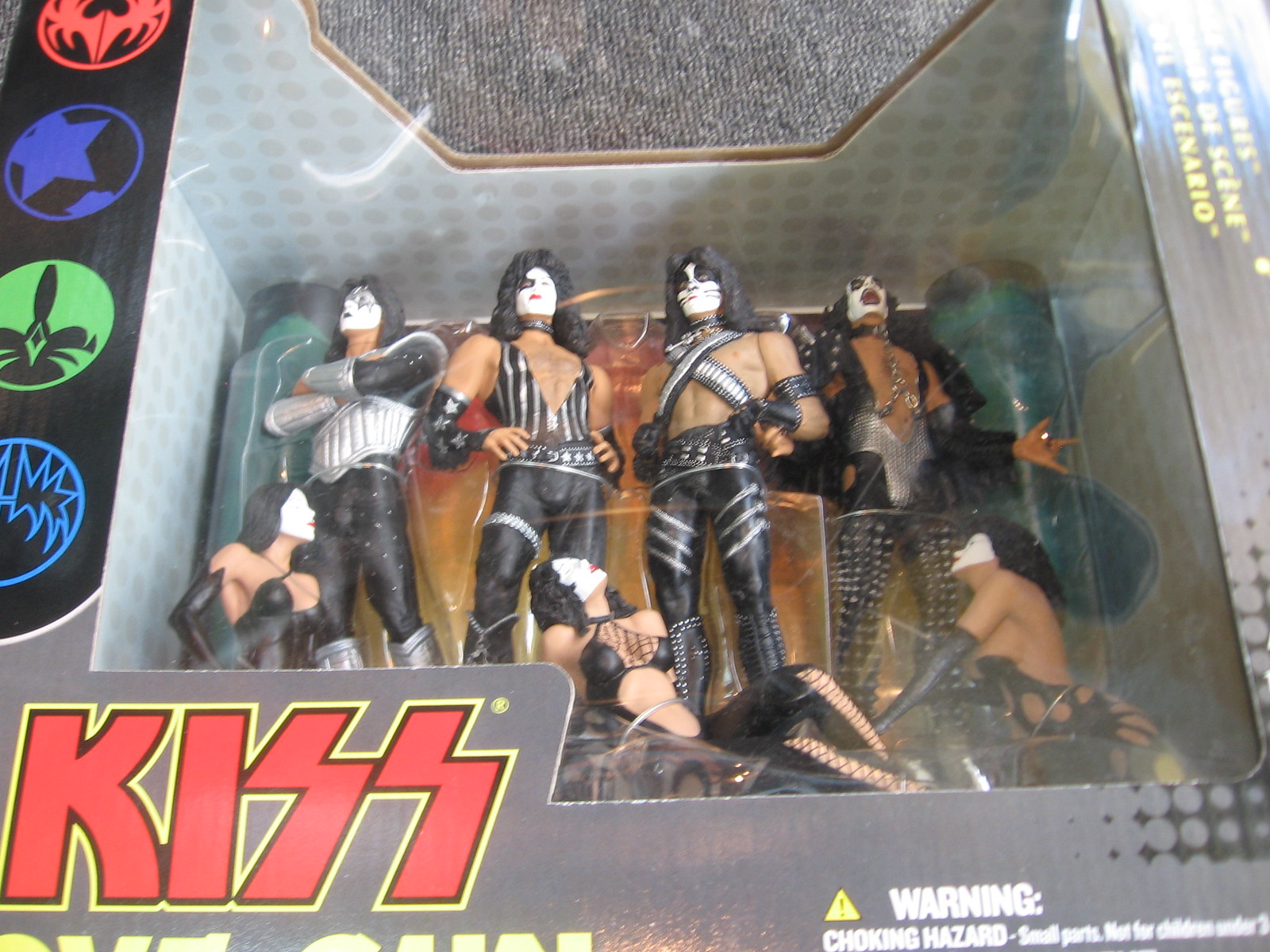The image shows a close-up, slightly blurred photograph of a collectible toy set featuring the rock band KISS in figure form. The boxed set, viewed from a top-down angle, occupies most of the image, with a small section of gray carpet visible through a cutaway at the top center. The box displays the large red KISS logo in the bottom left corner with some yellow text underneath, though the latter is difficult to read. To the right and up the side of the packaging, the gray cardboard continues, with colorful symbols in blue, green, purple, and red ascending on a black background along the left side.

Inside the unopened box, protected by a clear plastic window, are seven action figures. The four male band members stand prominently, adorned in their iconic black leather jumpsuits and signature face paint. Surrounding them are three scantily clad female figures, lounging provocatively at the bottom of the box, dressed in black fishnet outfits that reveal a lot of skin, accessorized with chains and dog collars. The plastic packaging showcases the intricately detailed figures, recreating the theatrical essence of KISS. Additionally, a yellow warning sign in the bottom right of the box indicates "choking hazard, small parts not suitable for children under 3."